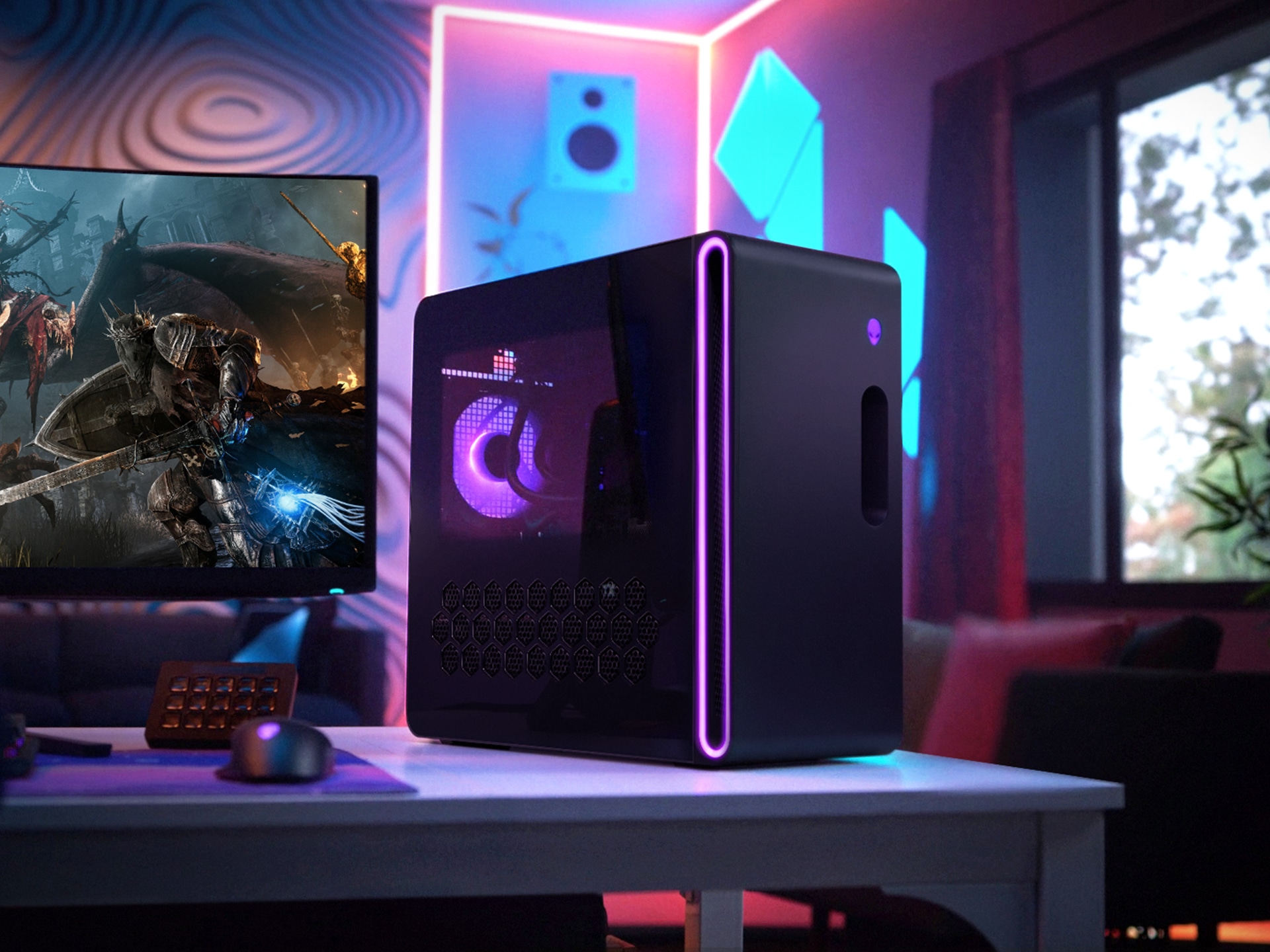This photograph showcases a high-end gaming setup in a dimly-lit room, suffused with a purplish hue from neon lights around the door, giving the space a futuristic ambiance. At the center of the image is a sleek black desktop computer, prominently displaying an alien logo which suggests it's an Alienware machine. This powerful-looking tower features purple lighting visible through its side panel, highlighting its advanced inner workings. It's mounted vertically on what appears to be a white desk, though the lighting makes the surface look purple.

To the left of the computer tower, there's a high-resolution monitor displaying a medieval-themed video game. The screen shows imposing knights clad in gray armor, wielding silver swords and shields, set against a backdrop of dragons and gray mountains with ancient-looking buildings. The monitor is thin with a black frame and partially shows a desktop speaker below it. A black mouse rests on a light and dark purple mouse pad, while a matching black keyboard lies nearby.

To the right of the setup is a window through which natural light streams in, illuminating green trees and casting intricate shadows on the lightly-colored walls. The room itself is adorned with vivid elements – the walls are described to have speaker-like designs in purple, complemented by turquoise shadows, and a blue-outlined speaker in the middle. There are also hints of decorative items, such as green and red pillows near the computer and what appears to be blue papers on the wall. This setup looks to be part of a personal office or den, perfectly tailored for an avid gamer.